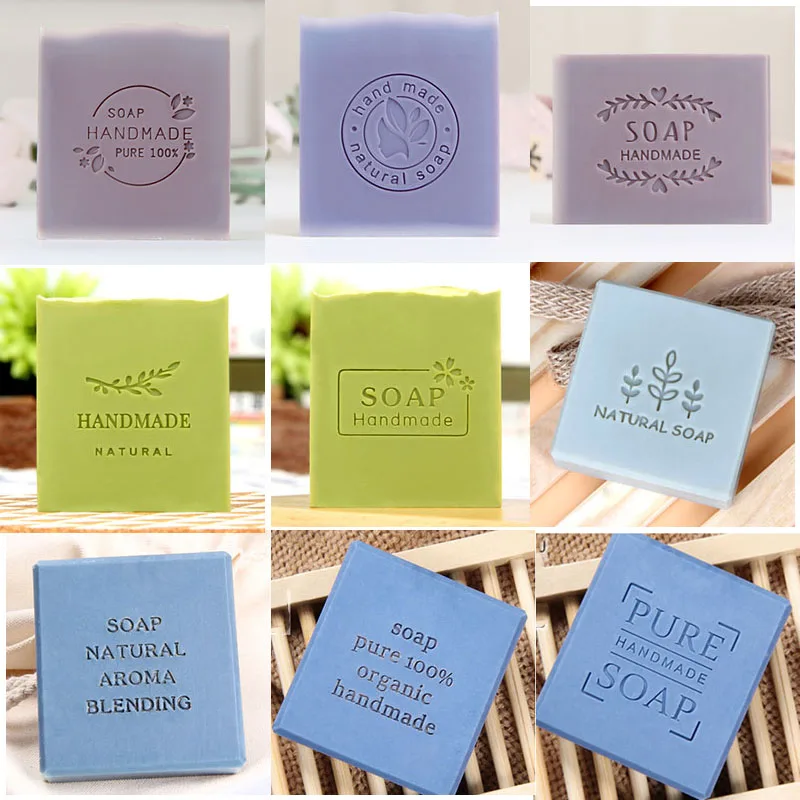This image is a detailed, vivid collage comprising nine separate photographs, each showcasing a square bar of handmade soap from a specific soap line. The collage is arranged in three rows and three columns, with each soap block featuring intricate designs or engraved text that highlights its handmade and natural qualities. The text includes phrases like "handmade soap," "natural soap," "100% organic," and "pure soap," emphasizing their artisanal and organic nature. The soaps display a vibrant array of colors ranging from purple, neon green, and blue to teal, yellow, and very light gray, presenting a visually appealing spectrum. These soaps are staged upright on a table, and the overall composition suggests a professional product showcase aimed at highlighting the variety and craftsmanship of the soap line.